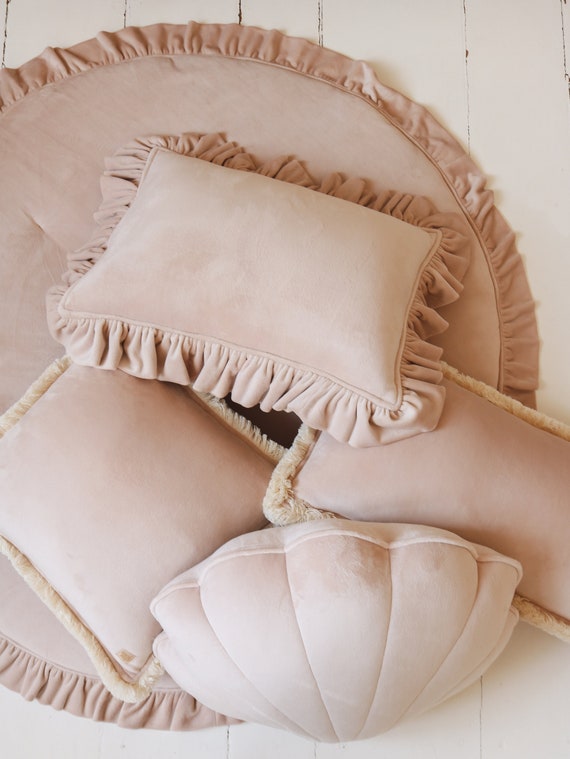This image features an arrangement of pillows in various sizes and shapes meticulously placed on a white wooden bench. Against the wall, you can observe white-painted wooden slats adding a rustic yet clean background to the scene. The bench seat also consists of these white wood planks, creating a harmonious and cohesive setting.

The pillows themselves are predominantly a creamy beige tone, blending seamlessly with the serene, monochromatic environment. In the background, a large round pillow adorned with decorative fringe takes center stage. In front of it, several smaller square pillows come into view; one of these square pillows shares the same type of fringe detailing, while the other two are bordered by a softer material, lending a touch of textural variety.

Additionally, there are three smaller pillows of diverse shapes—circular and rectangular—interspersed among the larger ones. In the forefront, a uniquely shaped pillow resembling a seashell stands out, adding a whimsical and naturalistic element to this tranquil and inviting setup.